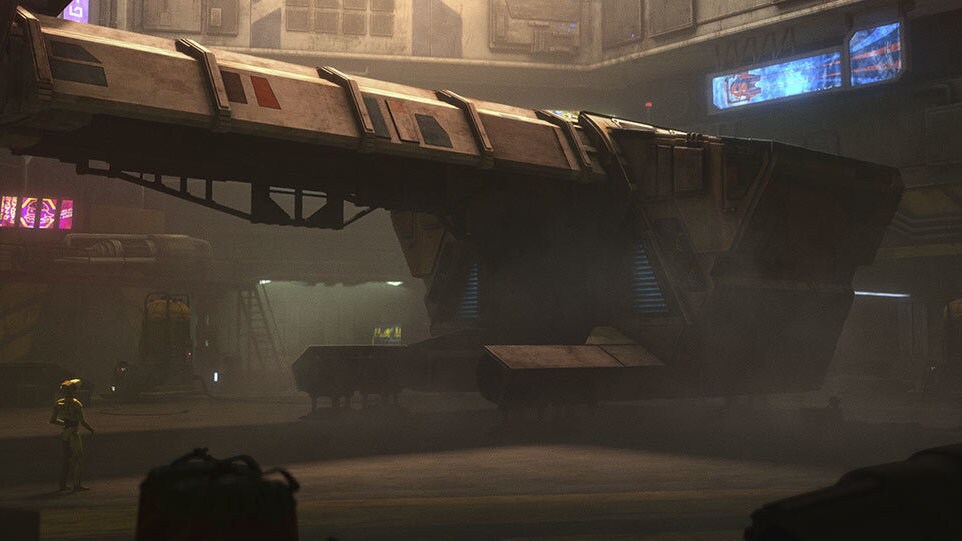In a dimly lit, smoky garage, an elongated sci-fi spacecraft with a pointed nose, main body, and two air blasters hovers ominously. The scene is shrouded in haze and darkness, reminiscent of a Star Wars landing bay. Surrounding the vessel are multiple video screens—blue ones on the upper right and pink ones on the left—casting an eerie glow. On the ground in front, either a robot or a small green alien stands, gazing up at the machinery. The gritty, industrial atmosphere is punctuated by a large window with multiple panes and vents at the top level. This futuristic and cluttered setting could be straight out of a movie or a themed attraction at a place like Disneyland, with its entrancing blend of technology and otherworldly elements.